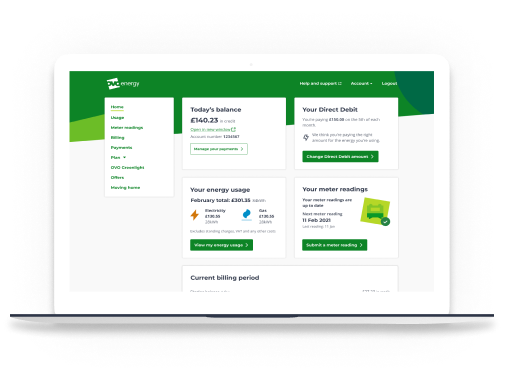In this image, a laptop screen displays a detailed energy usage dashboard. The interface showcases various sections including DVD Energy, Home Usage, Interior Reading, and a TV segment. Further down, it provides information on Interior Readings, Billing, Payments, and Plans. Highlighted are options for DVO Cross Lights and Special Offers. Noteworthy figures include today's balance of £140.23 and a total energy usage cost of £301.35 for February. The screen confirms that meter readings are up to date, with the next reading scheduled for 11 February 2021. Additional options allow the user to submit a meter reading or view detailed energy usage data for the current billing period.